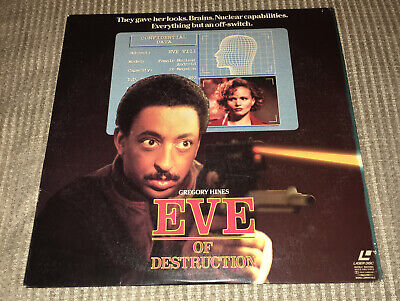The image appears to be a Laserdisc cover for the movie "Eve of Destruction," prominently featuring Gregory Hines. The cover rests on a beige woven fabric. At the top, there is a blue rectangular graphic with a computer-generated profile of a head, exhibiting horizontal and vertical grid lines. Below this, there's a photograph of a woman with short curly reddish hair gazing to the left. Above this blue rectangle, bold text reads, "They gave her looks, brains, nuclear capabilities. Everything but an off switch." In large red letters, the title "Eve" is capitalized and underlined, followed by "of Destruction." Gregory Hines, appearing in the central left of the image, is depicted with short hair and a mustache, holding a laser gun with both hands. Yellow laser beams are shown emanating from the gun. The overall composition of this movie poster emphasizes Hines' intense focus and readiness, further accentuated by his direct stare to the right. On the bottom corner, there's a small Laserdisc symbol.